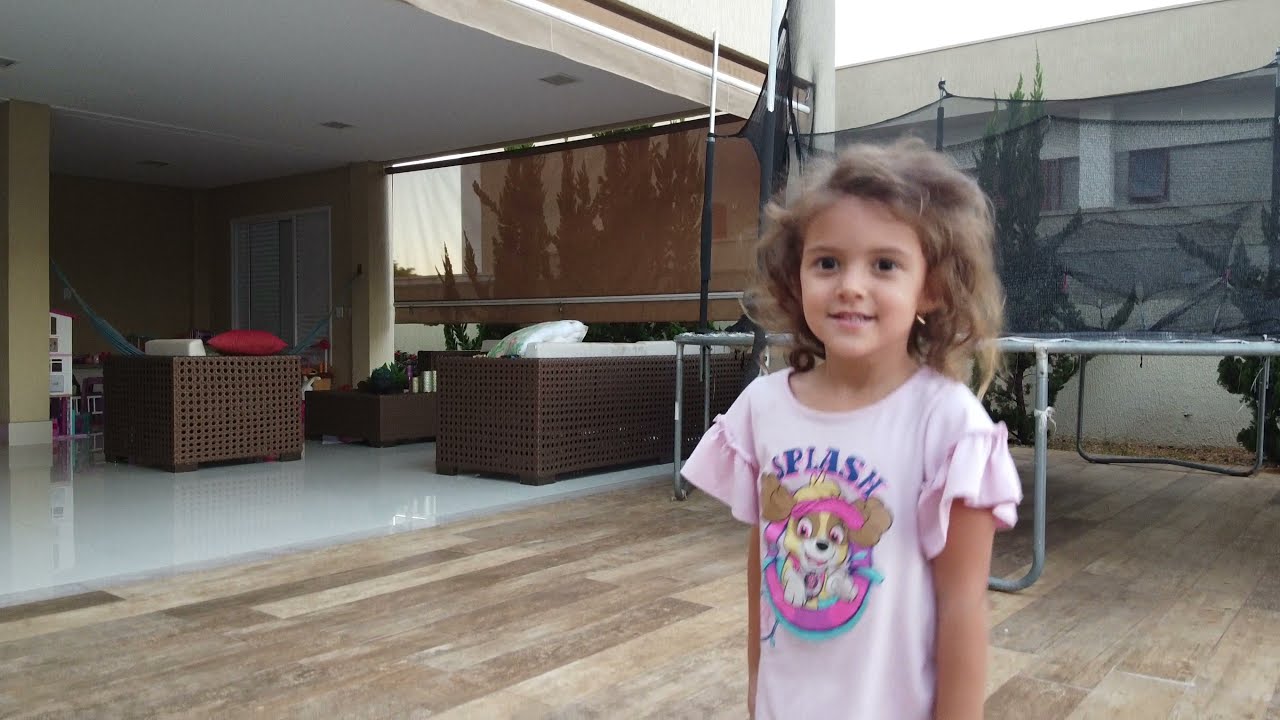The image features a very young girl, likely around six or seven years old, who is smiling directly at the camera. She has blonde hair, which appears to be slightly tousled as though from a breeze. The girl is wearing a pink t-shirt that features a cartoon picture of a beagle dog wearing a pink visor, with the word "SPLASH" written above it in blue letters. Her arms are relaxed and hanging down by her sides.

The girl is standing on an outdoor wooden slat floor, which resembles a patio deck. To the right behind her, there is a trampoline with metal legs and black safety netting. The background includes a partially enclosed patio area with dark brown wicker furniture arranged under a ceiling cover, and the floor beneath this covered area is made of shiny white material. Further to the left in the image, there is what appears to be a stairway leading to a second floor and a screen, possibly for tennis, suggesting the presence of a tennis court nearby. The overall setting is outdoors on what appears to be a cloudy day.